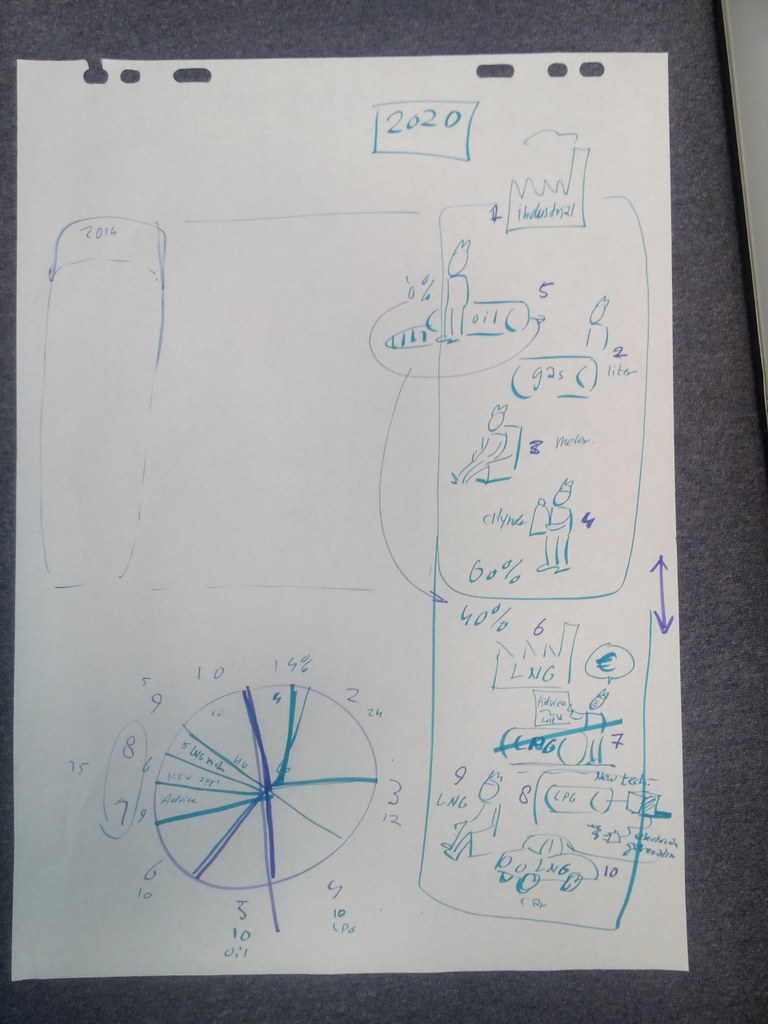The image depicts a white sheet of paper clipped onto a black clipboard, covered with a mixture of doodles and mathematical or assignments-related notes drawn with a blue pen. At the top of the sheet, enclosed in a box, there is writing that includes the year or number "2020." On the right side, there is a series of small panels featuring a figure in various positions - standing, sitting, and standing again - along with a sign labeled “gas.” This sequence is vaguely thematic, suggesting some sort of narrative or instructional sketch. 

Adjacent to these panels, another box showcases percentages: "40%, maybe 60%," followed by "40%." There are illustrations of a bus and a car situated near these figures, adding to the image's complex yet unclear theme. The left side of the paper faintly reveals the year "2016," and beneath this, a diagram resembling a wheel is positioned, marked with numbers ranging from 1 to 10. Each of these numbers is accompanied by pie-chart-like segments.

Overall, the image appears to be an eclectic blend of casual doodling and structured notes, possibly related to a homework assignment or mathematical work.